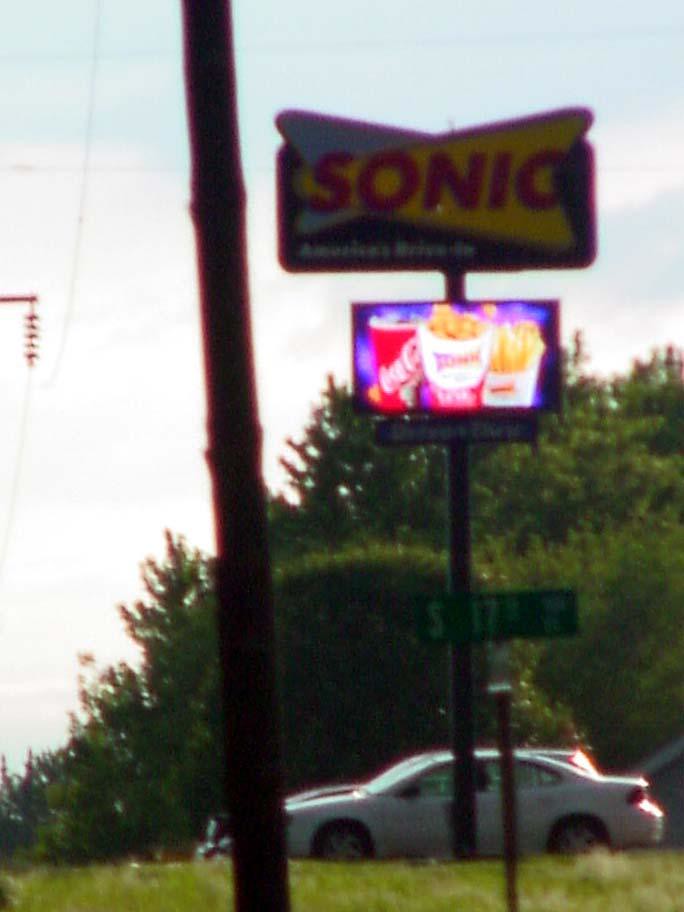This image features a slightly blurry and out-of-focus view that appears to be taken from the side of the road. Dominating the scene is a prominent SONIC fast-food restaurant sign with bold red letters set against blue and yellow backgrounds. Directly beneath this main sign is a digital display showcasing a cup of Coke with a red background and white letters, alongside some yellow French fries in white packaging, and an unidentified item in white packaging. To the left of the sign stands a brown telephone pole supporting electrical wires that stretch across the upper part of the image. Below the Sonic sign, there's a green street sign with white letters spelling out S17. The bottom part of the image includes a patch of grass and a grey car. In the background, there are scattered green trees and a clear blue sky dotted with a few white clouds.